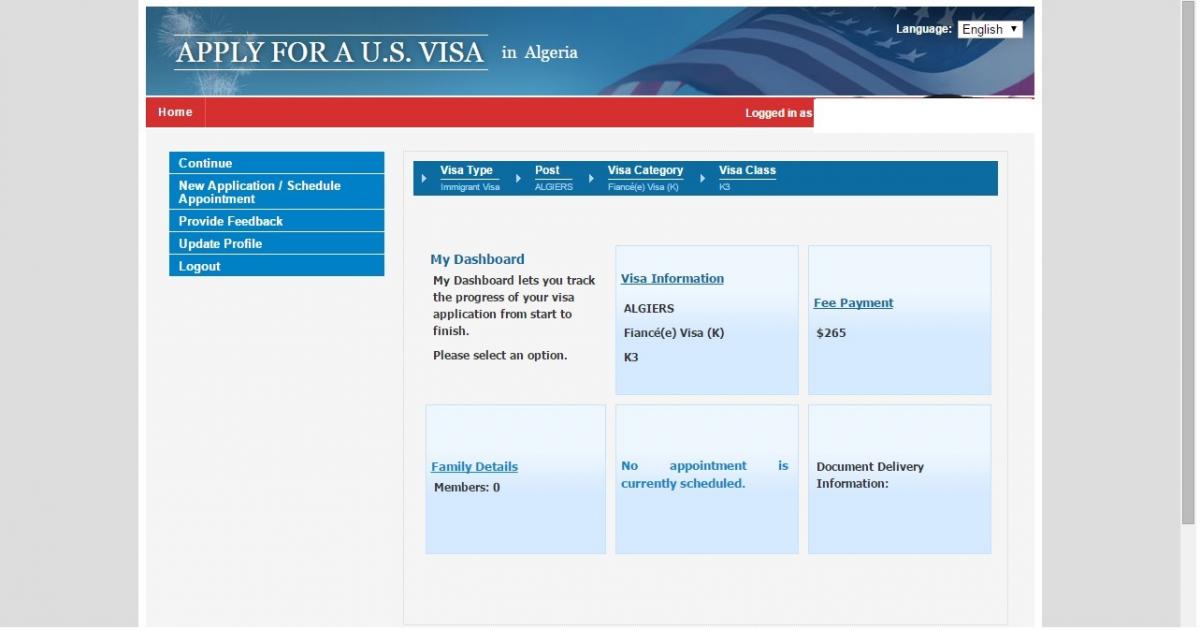The primary background of this webpage is light gray, accented by a white border framing the top portion. Prominently featured is a banner depicting the American flag waving in the wind on the right side, rendered with a curved motion line to emphasize its movement. To the left of the flag, wispy white shapes hint at clouds in the sky. Below the banner is a white line, followed by bold, all-capital text in a Georgia font that reads "APPLY FOR A U.S. VISA." This headline is in large lettering, and another white line sits beneath it for emphasis. In smaller white capital letters under the headline, it states "IN ALGERIA."

In the upper right corner, there is a bold label in small white text that says "LANGUAGE:". Next to this is a dropdown menu, designed as a white rectangle displaying the word "ENGLISH" in black text, accompanied by a black arrowhead icon indicating the menu can be expanded.

On the left of the webpage is a horizontal navigation bar. The majority of this bar is red, but about one-third is white. On the red section, the word "HOME" appears in white text on the left side. To the right, within the white section, it says "LOGGED IN AS," but the user’s name or username is obscured by a white rectangle to maintain privacy.

Below this horizontal bar, on the left side of the page, is a vertical menu set against a medium blue background. The menu options are listed in small, bold white text, each separated by a thin white line. The options available are "CONTINUE," "NEW APPLICATION / SCHEDULE APPOINTMENT," "PROVIDE FEEDBACK," "UPDATE PROFILE," and "LOG OUT."